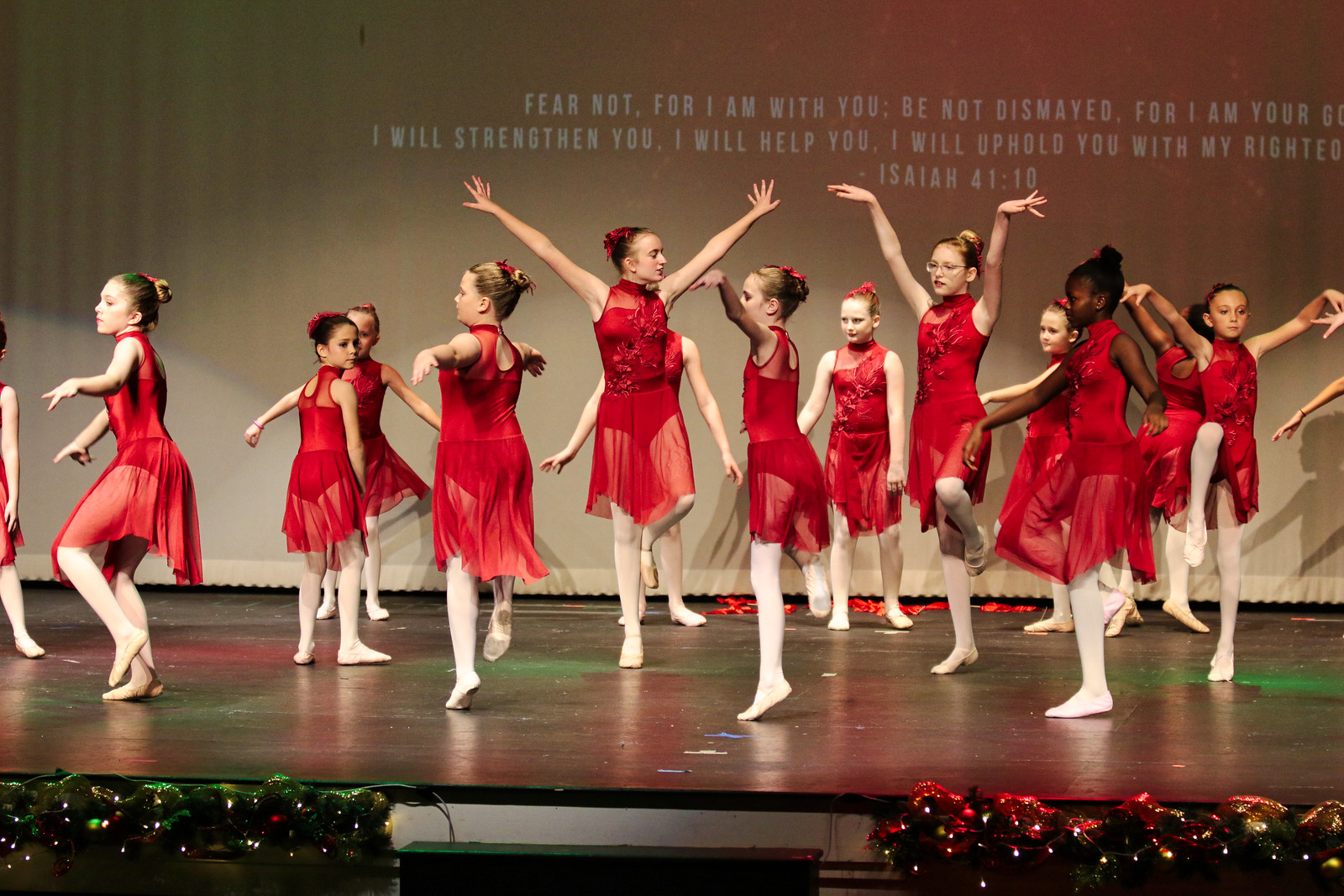A group of approximately 12 to 15 young girls, predominantly white with at least one Black girl visible, are performing a ballet dance on a black stage adorned with Christmas lights — green on one side and red on the other. They are all dressed in elegant red dresses with frilly bottoms, paired with ballet stockings and shoes. The girls are in various ballet poses, some with arms raised and others with arms down or legs up, and their hair styled in neat buns. The stage background features a brown curtain with a prominently displayed quote in white lettering: "Fear not, for I am with you. Be not dismayed, for I am your God. I will strengthen you. I will help you. I will uphold you with my right." The verse, attributed to Isaiah 41:10, provides a powerful backdrop to their performance. In addition to the lights, there is a speaker placed between the lights in front of the stage, enhancing the festive atmosphere.